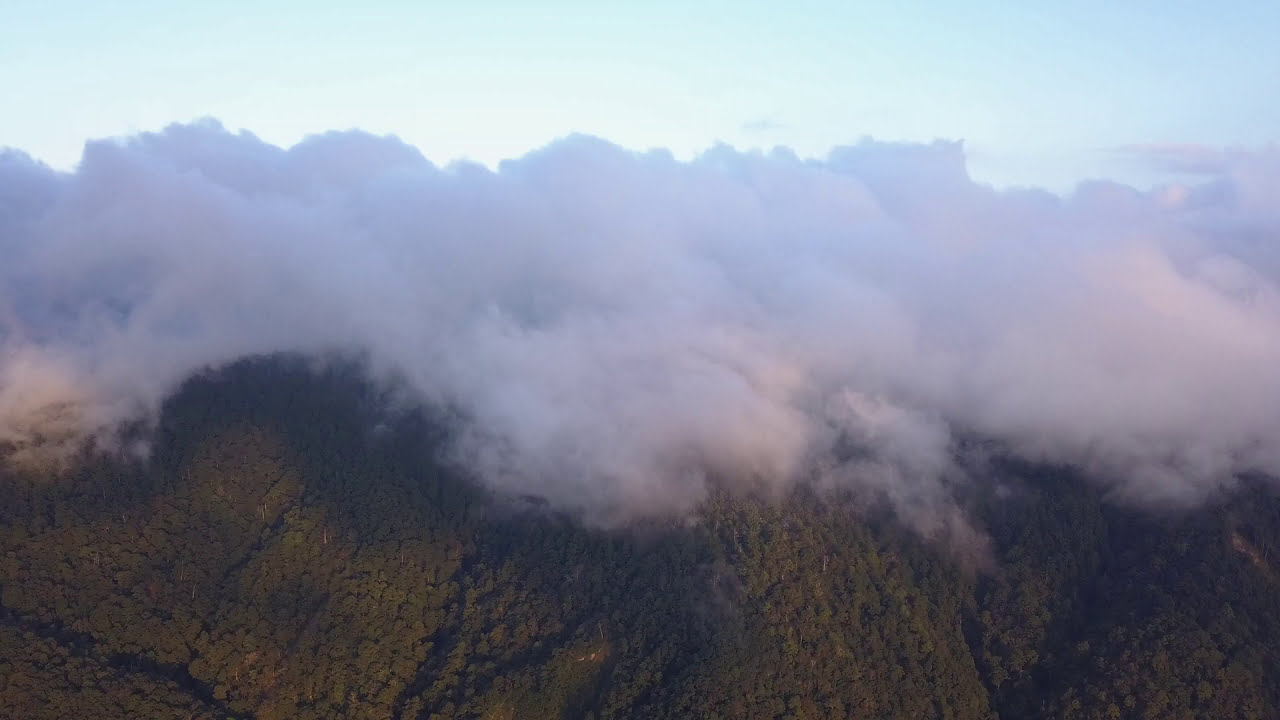This color photograph, taken from a high vantage point using a drone, beautifully captures a densely forested mountain range enveloped in a shroud of light gray, mist-like fog. The photo, in landscape orientation and representational realism style, presents a striking contrast between the lush green canopy of trees densely packed together on the mountainsides and the pale blue, cloudless sky above. The line of thick fog spans horizontally across the middle of the image, obscuring the mountain tops and creating an ethereal barrier between the vivid greenery below and the expansive sky above. The image is detailed enough to discern individual trees, though their leaves remain indistinguishable due to the height from which the photo was taken, likely several hundred feet above the mountains.